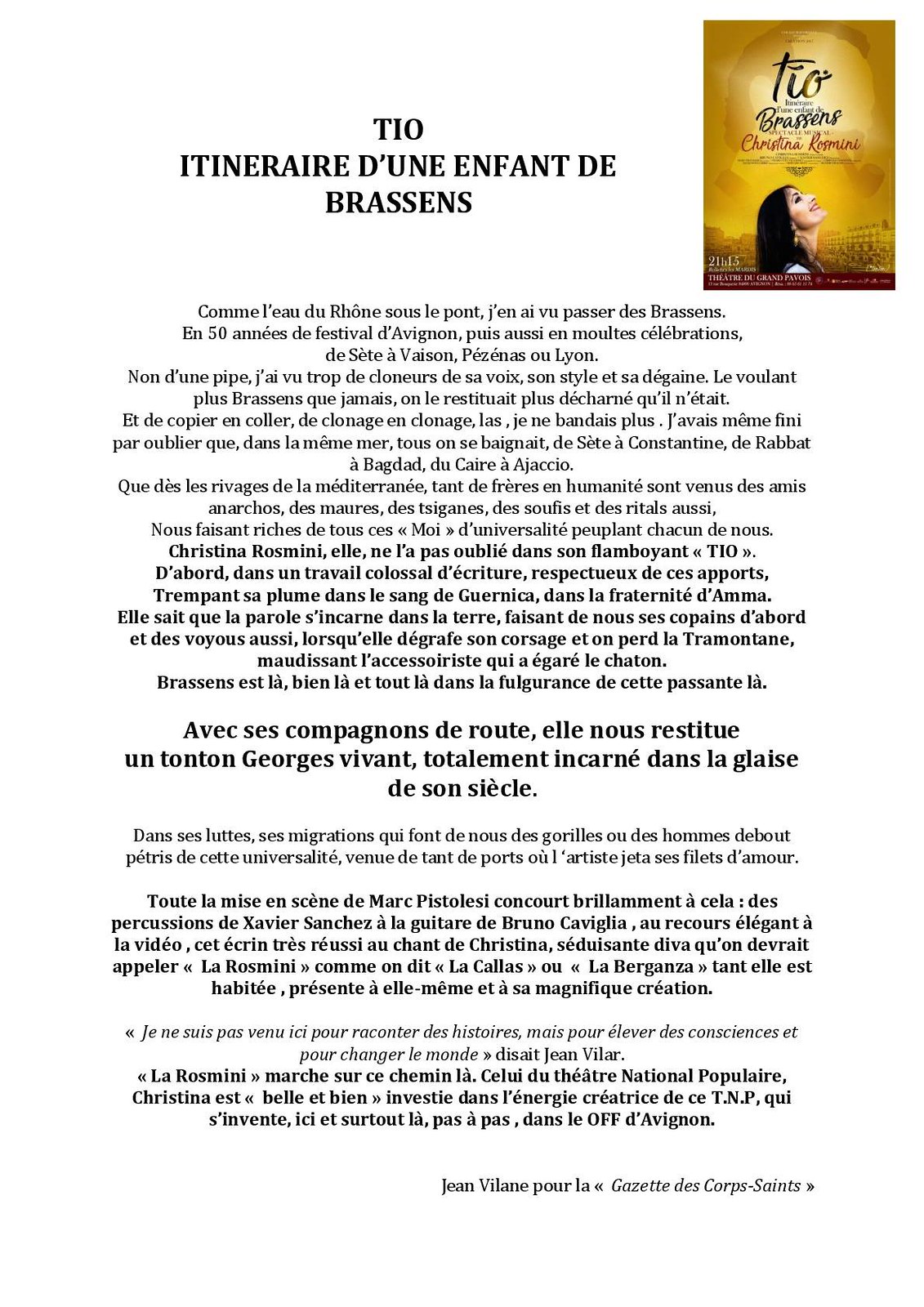The image showcases a detailed page of text in a foreign language, likely French, with a headline titled "T.I.O. Intenerere D-U-N-E" and "D. Brasens" at the top. This text appears to be an advertisement for a play, musical, book, or DVD, executed in black font on a white background. Prominent in the upper right corner is a small, gold-toned display image labeled "T.O. Rosen's Christina Rosmini." The name Rosmini, depicted in smaller text, features Christina Rosmini, a woman with long black hair gazing upwards towards the sun. In this visual, she is situated against a background that suggests a bustling marketplace or plaza with visible buildings. Additionally, there is an image portraying a man smoking a pipe. At the bottom of the page, the script is signed with the name Jean Villan-Pourla, associated with the "Gazette des Corps Saints," thus offering a comprehensive descriptive advertisement that blends text and imagery to suggest an artistic or cultural media piece.